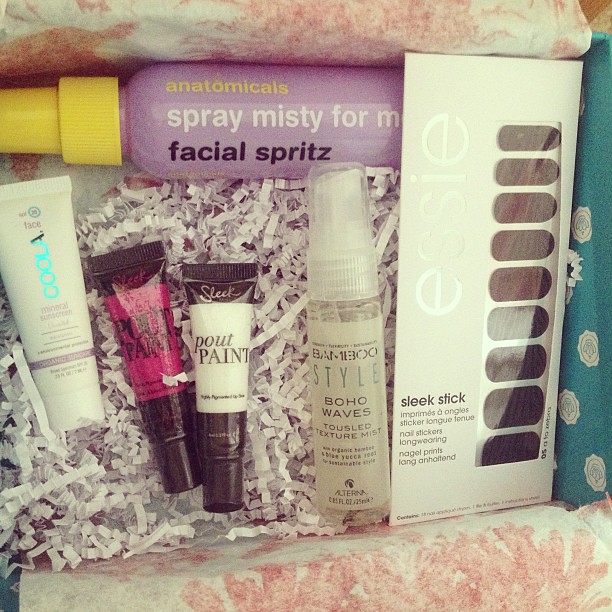In this image, a decorative box filled with crinkled paper shreds and makeup items is displayed. At the top of the image, there's a spray pump bottle with a yellow cap and a pink body, labeled "anatomicals, spray misty for me, special spritz." Below this, we find four tubes: on the left, a white tube with the word "cooler" written in blue; next to it, a darker-colored tube labeled "pulse paint"; followed by another, similarly named "pulse paint," and lastly, a tube named "bamboo style boho waves." The box also contains an Essie Sleek Stick set for nail stickers and other colorful cosmetic items. The background features pink and white swirls with green sides and white decorative elements on them, adding a festive touch to the presentation.